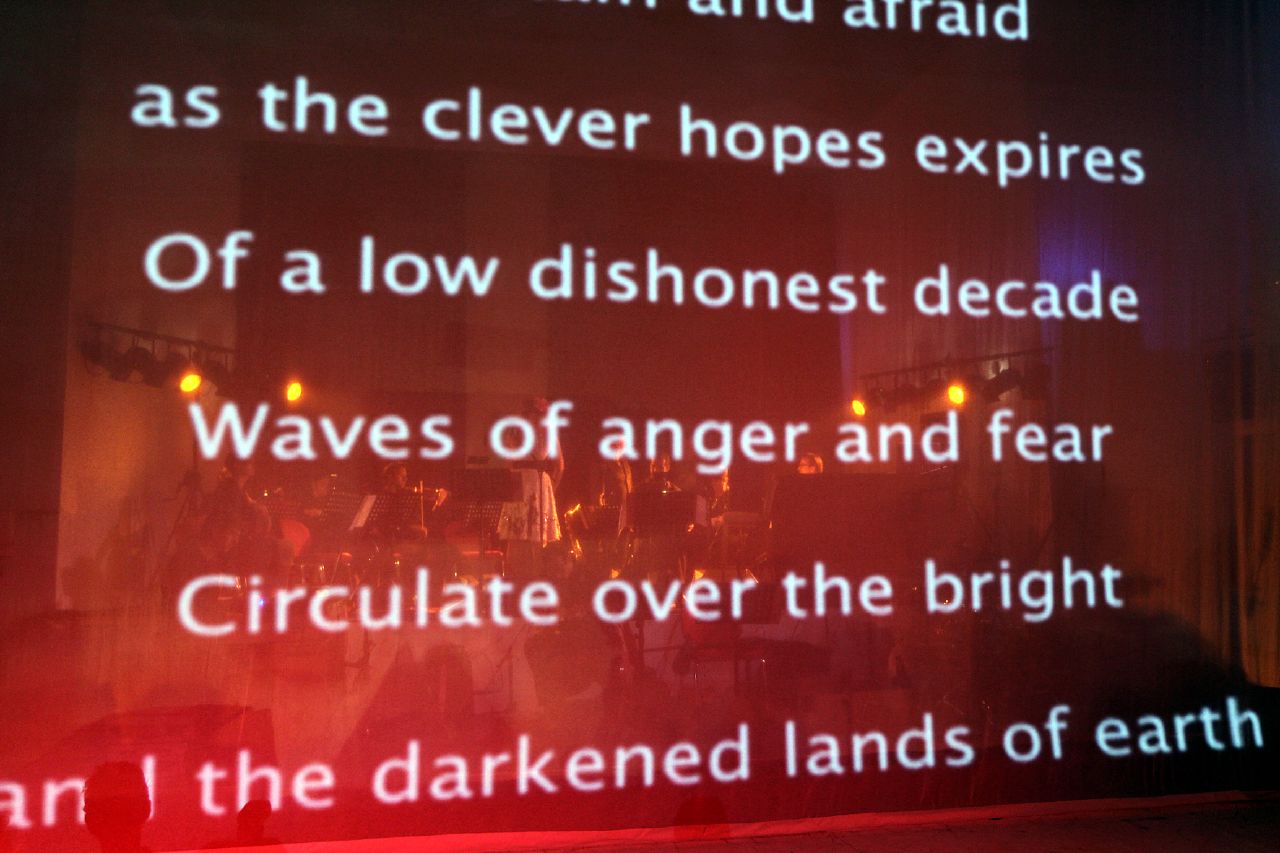The image depicts text with the prominent words: "Afraid as the clever hopes expire of a low dishonest decade, waves of anger and fear circulate over the bright and darkened lands of Earth." Though some text is cut off and difficult to read, there is a reflective overlay that shows a band playing. The reflection, likely from a window or glass, reveals a scene of about 15 band members under bright spotlights, with a female conductor in a white skirt leading them. The band is presumably facing an unseen audience. The lower left side of the text is partially obscured, possibly by a person.